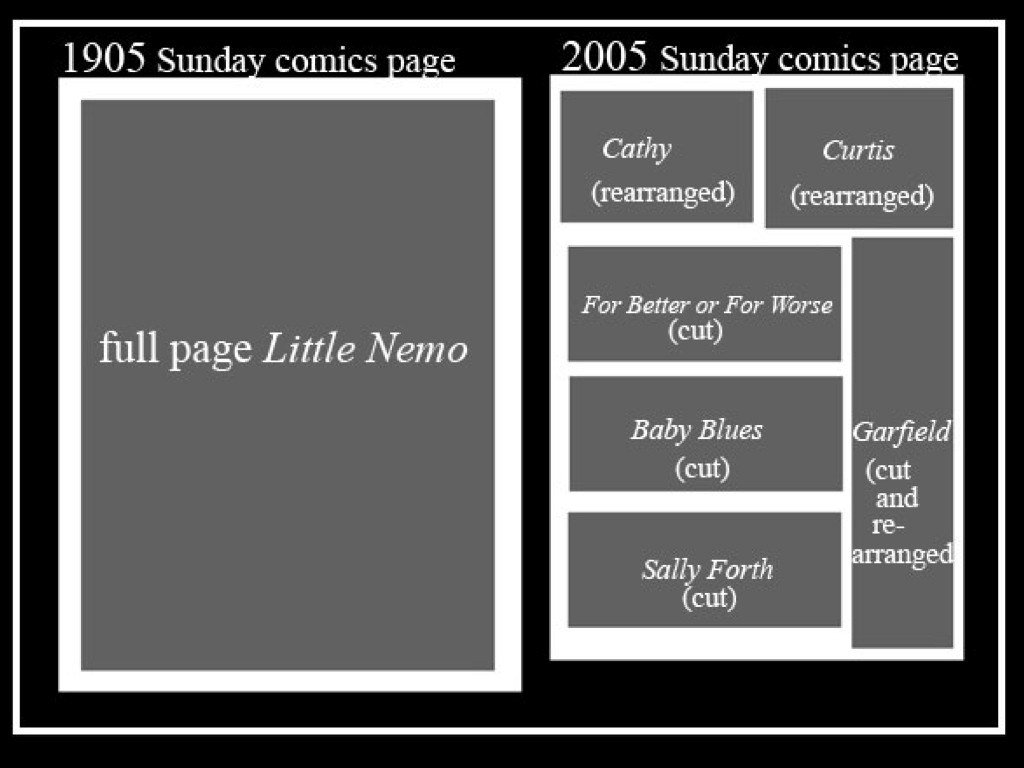The image features a black background with a white outer border. On the top left, there is a gray vertical rectangular section framed with thick white lines. Above this section, it reads "1905 Sunday Comics Page" in white font, and within the gray area, it states "Full Page Little Nemo." Directly to the right, there is a smaller tall rectangular white frame segmented into several gray boxes. The header above this section reads "2005 Sunday Comics Page" in white font. Within the gray boxes, the captions in white font are as follows: "Kathy (Rearranged)," "Curtis (Rearranged)," "For Better or for Worse (Cut)," "Baby Blues (Cut)," "Sally Forth (Cut)," and a longer box spanning several smaller ones that reads "Garfield (Cut and Rearranged)."